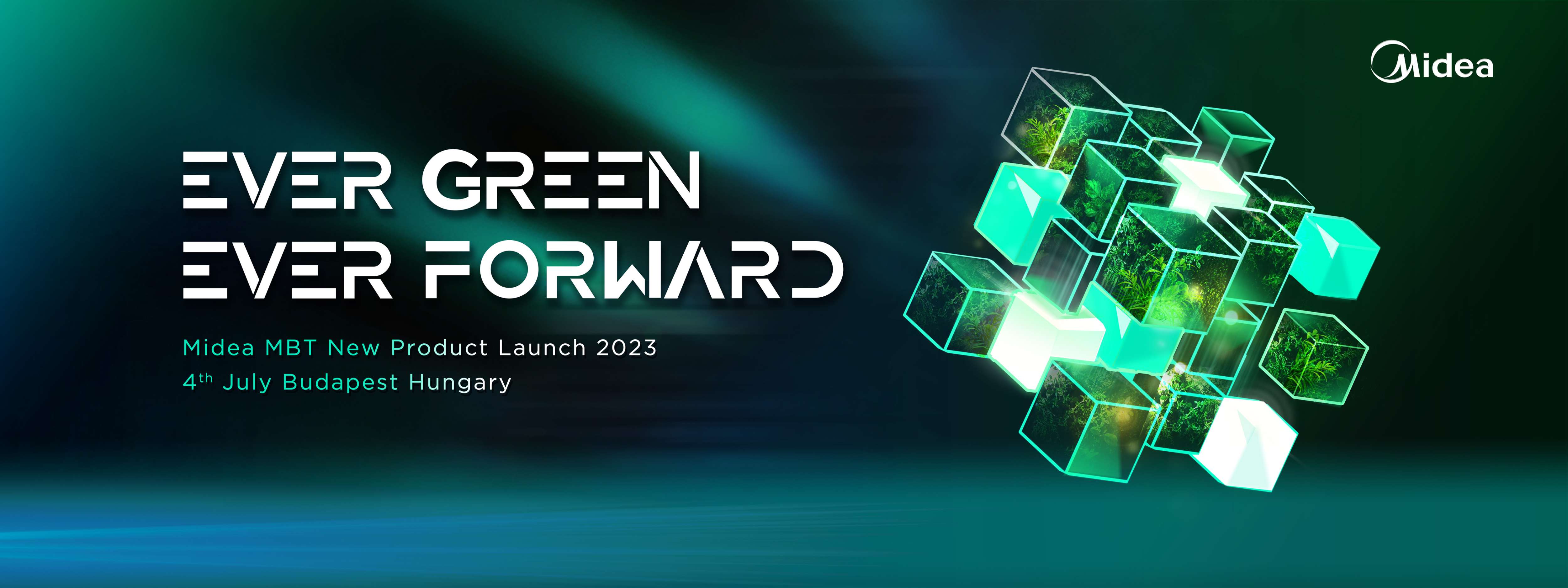The advertisement banner features a horizontally long rectangular image with a dynamic green-themed background that transitions from a lighter teal at the bottom to a darker green towards the top, incorporating light green streaks that evoke a northern lights effect. On the left side, prominent white text reads "Evergreen, Everforward," followed by smaller text detailing "MIDEA, MBT, New Product Launch 2023, 4th of July, Budapest, Hungary." The upper right corner contains the company logo, "MIDEA," encased in a bubble or globe-like circle around the 'M'. 

On the right side of the banner, a geometric array of cubes appears, resembling a disassembled Rubik's Cube. These cubes are closely clustered but not touching, creating a floating 3D effect. The cubes vary in appearance; some are white, some are a bright mint green with white triangles in their corners, and others are transparent containing hyper-realistic plants and ferns. The entire advertisement exudes a modern and technical aesthetic, highlighting the company's innovative image and new product launch.